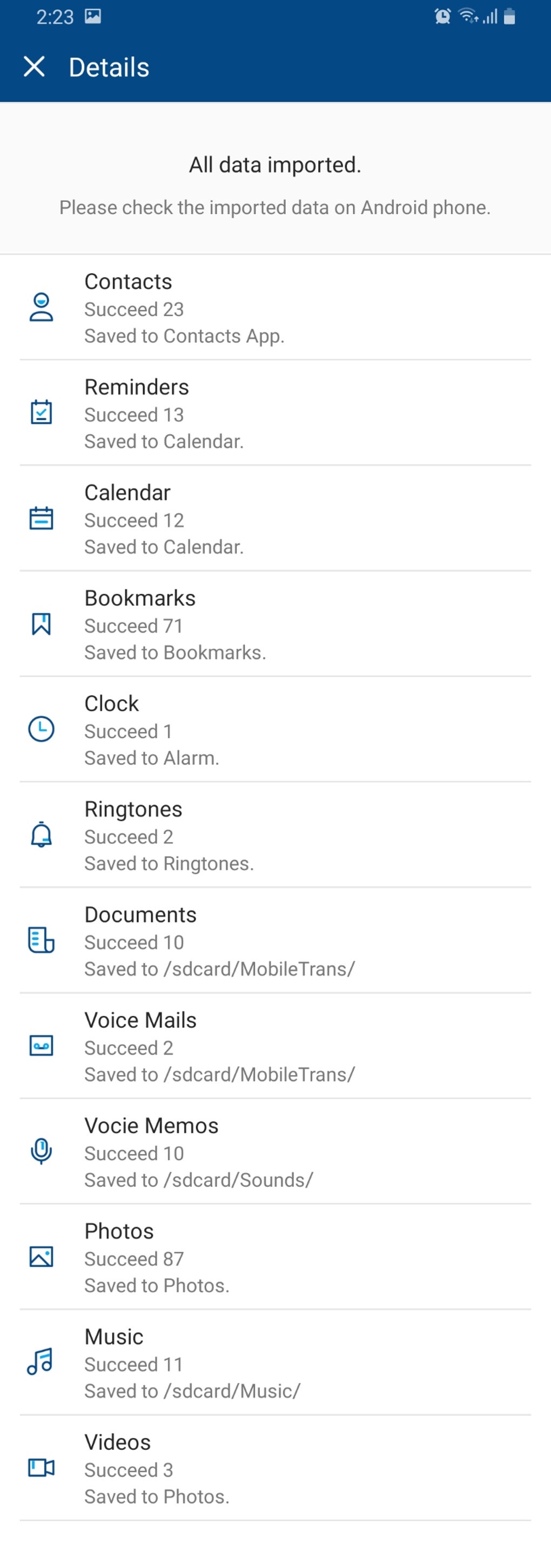The image appears to be a screenshot taken from a smartphone. In the upper left corner, the time is displayed as "2:23," accompanied by various symbols on the right side, including the internet and Wi-Fi icons. Below the time, there is an "X" button and a "Details" label in white text. Underneath this, the message "All data imported. Please check the imported data on Android phone" is displayed. 

The main portion of the screenshot shows a list of categories with corresponding icons and titles. Each item has a small icon on the left, followed by a title and some additional small text beneath.

1. Person icon: Contacts
2. Square with a checkmark: Reminders
3. Calendar icon: Calendar
4. Bookmark symbol: Bookmarks
5. Clock icon: Clock
6. Bell symbol: Ringtones
7. Paper icon: Documents
8. Square symbol: Voicemails
9. Microphone icon: Voice Memos
10. Photo icon: Photos
11. Music note: Music
12. Video camera: Videos

Each category appears to pertain to different types of data that have been imported, with small text details displayed underneath each title.